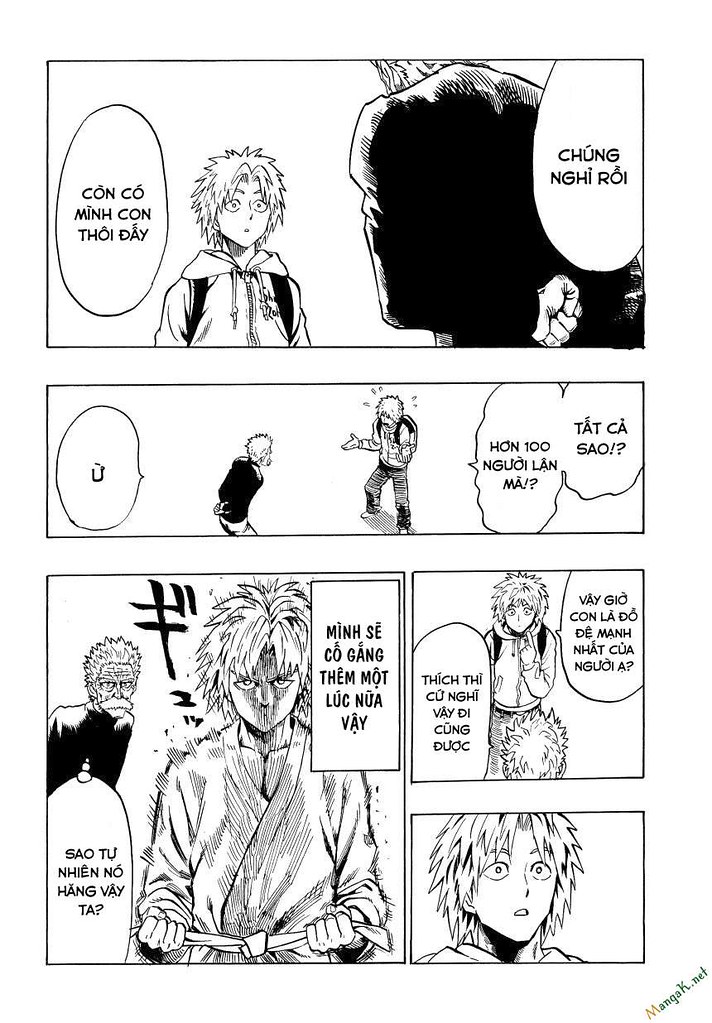In this black-and-white comic strip, likely from an Asian-inspired series and possibly in Vietnamese, the story unfolds across five distinct scenes. In the first panel, an imposing figure dressed in black, with his hands behind his back, speaks to a young, choppy-haired teenager wearing a hoodie. The teenager, whose name appears to be Trung Duy Huy, looks nervous. In the following panel, the man in black raises his voice, and anger marks emanate from the teenager's head as he responds with frustration. The focus then shifts to the bottom left panel, where the teenager has donned a karate outfit and is tightening his belt, displaying newfound confidence. The man, seemingly named Sau Tu Huynh Ngo Vinh Ve Top, observes him with a mix of surprise and contemplation. In the next scene, the teenager is back in his hoodie, resuming a dialogue with the figure in black. The concluding panel shows the teenager deep in thought, suggesting contemplation or a sense of resolve after the exchange.